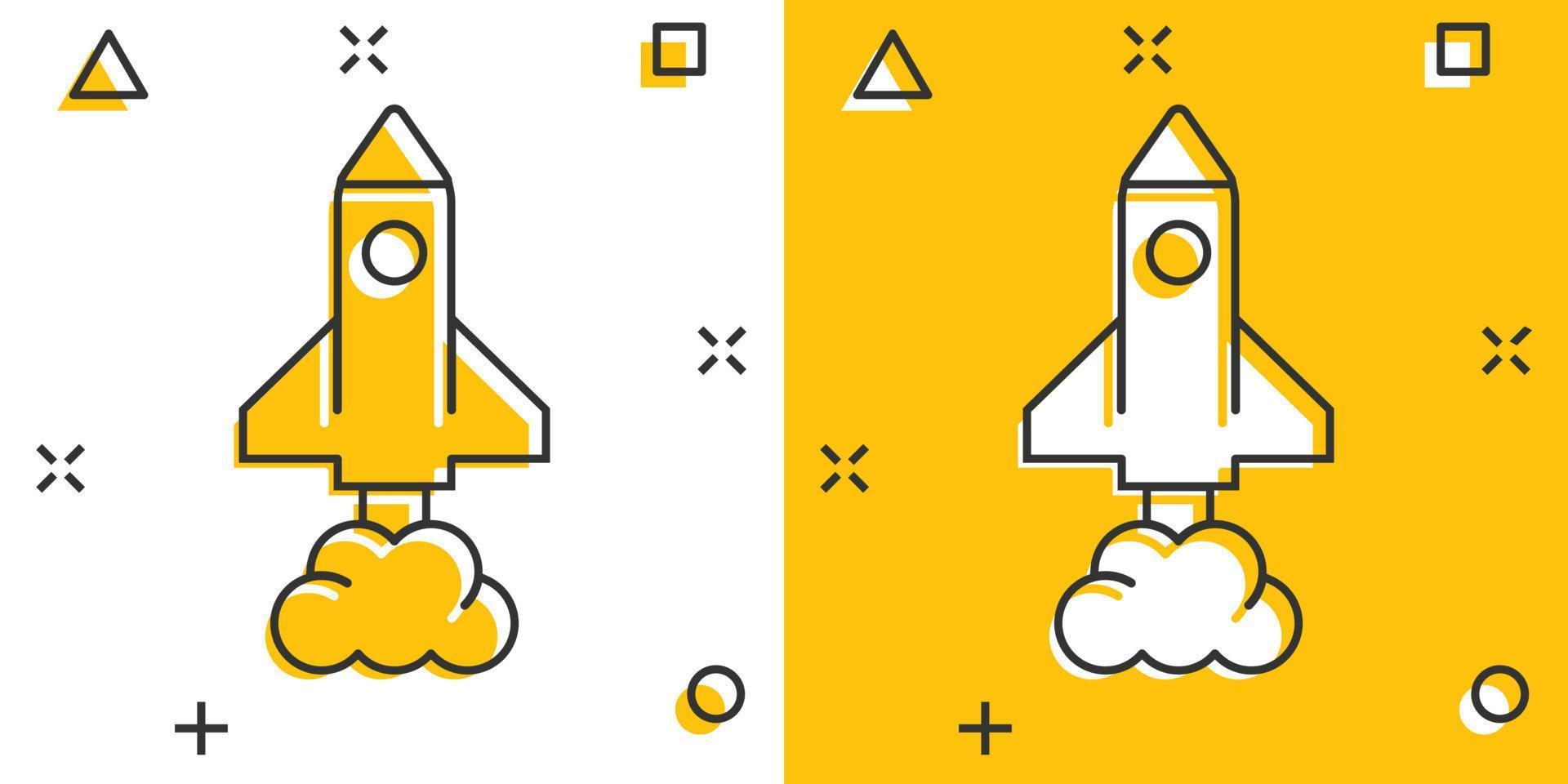This image features two clip art-style rocket ships positioned side-by-side, each drawn with minimalist, straightforward lines. On the left side, a mustard-yellow rocket sits on a stark white background, while on the right side, a white rocket appears against a mustard-yellow backdrop. Both rockets are nearly identical, featuring a simple circular window near the top and small clouds at their bases, indicating they are launching.

Arranged around each rocket are four geometric symbols – a triangle in the top left corner, a square in the top right, a circle in the bottom right, and a plus sign in the bottom left. These elements, reminiscent of PlayStation console symbols, are precisely positioned in the same locations on both sides.

The entire composition is rendered in a style that combines bold black outlines with slightly offset colors, giving the image a graphic design aesthetic. This visual effect adds depth and a subtle sense of dimension. The simplicity of the design, with limited lines and shapes, lends itself to varied applications, making it suitable for everything from children’s decor to potential advertisements. 

Three small stars are sprinkled on both sides of the image, adding a whimsical touch. Overall, the alternating color scheme and the neat arrangement of shapes result in a balanced, eye-catching graphic.